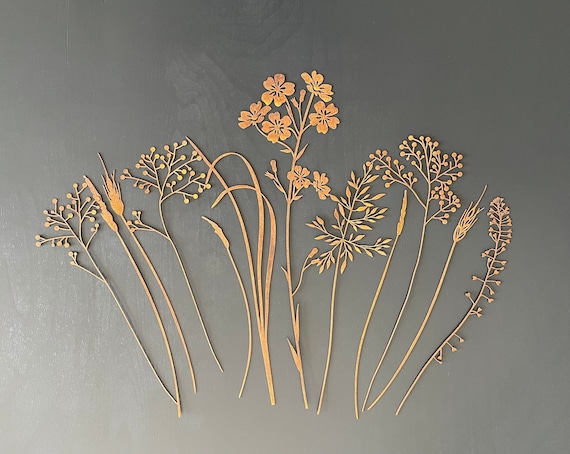This image depicts an artistically arranged collection of botanical elements against a gradient gray background that fades from dark at the top to lighter at the bottom. At the center of the composition, several tall and elegant stems showcase large, beautiful flowers in a light orange color, standing out prominently. Surrounding these central blooms, there are various other plant shapes, including different kinds of leaves and smaller flower buds. The plants appear to be either artistically crafted cutouts or meticulous drawings, and they are arranged in a way that some stems are curved and some are more upright. The additional elements, like delicate wheat stalks and wildflower sprigs, create a scene reminiscent of a natural grassy plain, with various leaves and miniature flowers still in bud. Overall, the image presents a harmonious and detailed botanical display, all uniformly colored in light orange tones, set against a thoughtfully shaded gray backdrop.